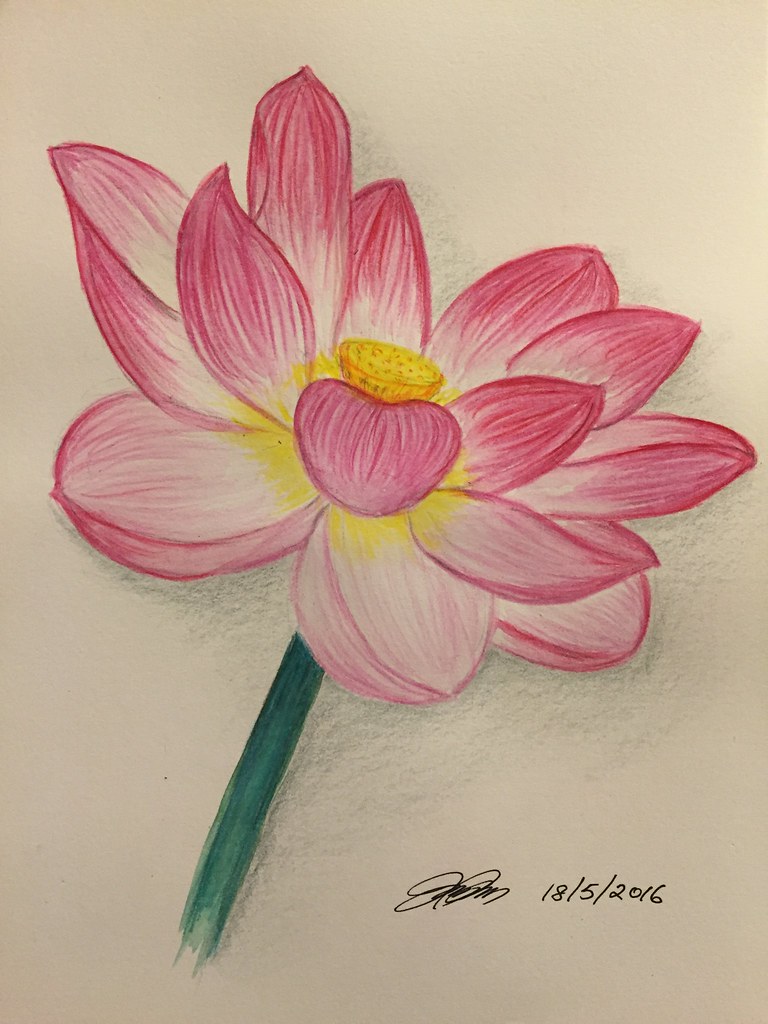This image features a detailed drawing of a lotus flower on cream-colored paper. Dominating the center of the image is a large, vividly colored lotus with a deep green stem that points slightly towards the lower left corner. The petals, shaded in gradients of pink and reddish tones, emphasize texture and depth, with a bright yellow center that subtly bleeds into the bases of the petals. The artist has employed skillful shading techniques, using both graphite and colored elements to portray lighting and depth. In the bottom right-hand corner, there is an artist's signature and the date, somewhat hard to decipher, but marked as May 18th, 2016. The drawing stands out for its artistic detail and use of color, giving the flower a striking, visually dynamic quality.